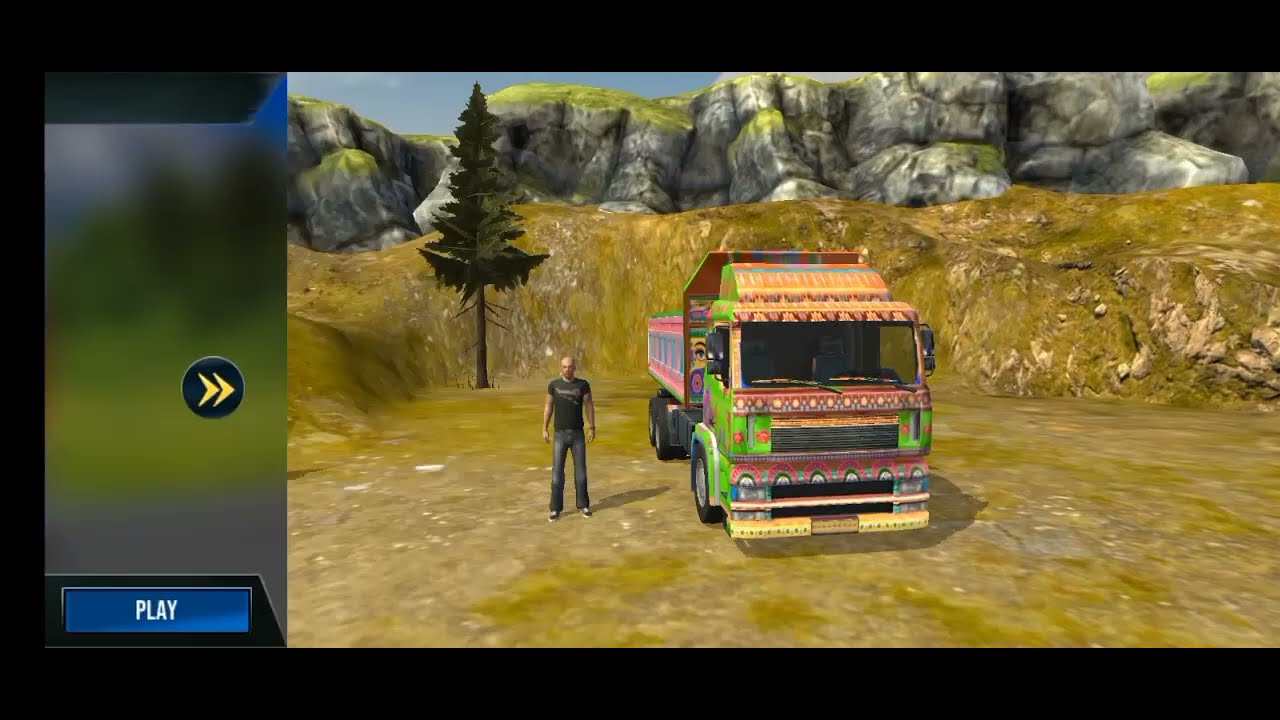The image is a detailed screenshot from a video game, featuring a vibrant, multicolored dump truck parked on a rocky, grassy terrain. The dump truck stands out with its unusual, tricked-out paint job that incorporates bright neon greens, oranges, bubblegum pinks, purples, and stripes, as well as floral patterns. Beside the truck, slightly behind the passenger side door, stands a bald man with a light skin tone, wearing gray jeans, a black short-sleeved t-shirt with white lettering, and black sneakers with white soles and laces. His body is relaxed with arms at his sides. The background showcases a rugged mountainous environment with brown rock formations, some covered with moss and scattered vegetation, and a solitary pine tree. In the left-hand corner of the screenshot, there is a black circle with two yellow arrows pointing to the right and, below it, a blue rectangle displaying the word "PLAY" in white text.